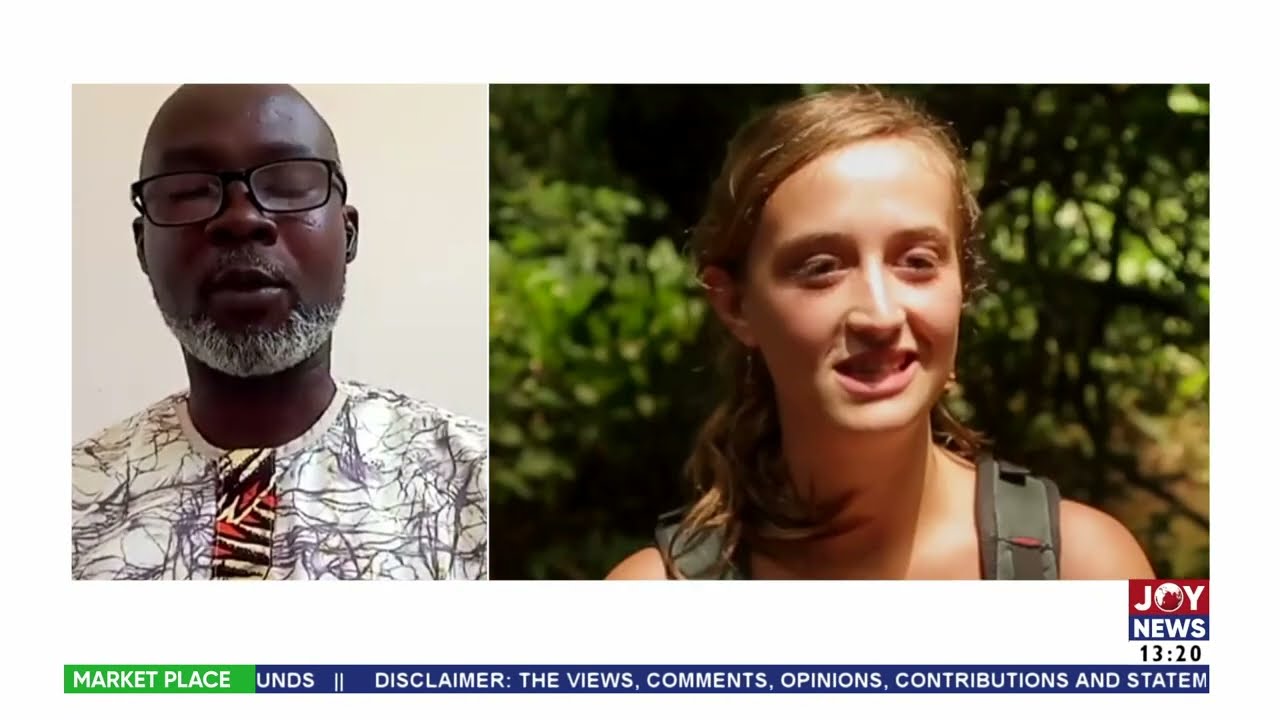The image is a TV news screenshot featuring two individuals. On the left, there is a dark-skinned man with a gray beard and black glasses. He is dressed in a light-colored shirt with a design comprising of white, black, orange-red, and gray elements, resembling an African-style garment. His image occupies about one-third of the screen. On the right, a young white woman with blonde hair that falls over her shoulders is seen smiling and looking slightly to the right. She appears to be a backpacker, as she is wearing a backpack with green straps and has a green leafy background behind her. Her image takes up roughly two-thirds of the screen. At the bottom right of the screen, a black rectangle displays the "Joy News" logo, with the "O" depicted as a globe and the current time of 13:20. Beneath this is a banner with white text on a blue background that reads, "Marketplace," followed by a disclaimer stating, "the views, comments, opinions, contributions, and statements." The overall design suggests a news program segment featuring these two individuals.